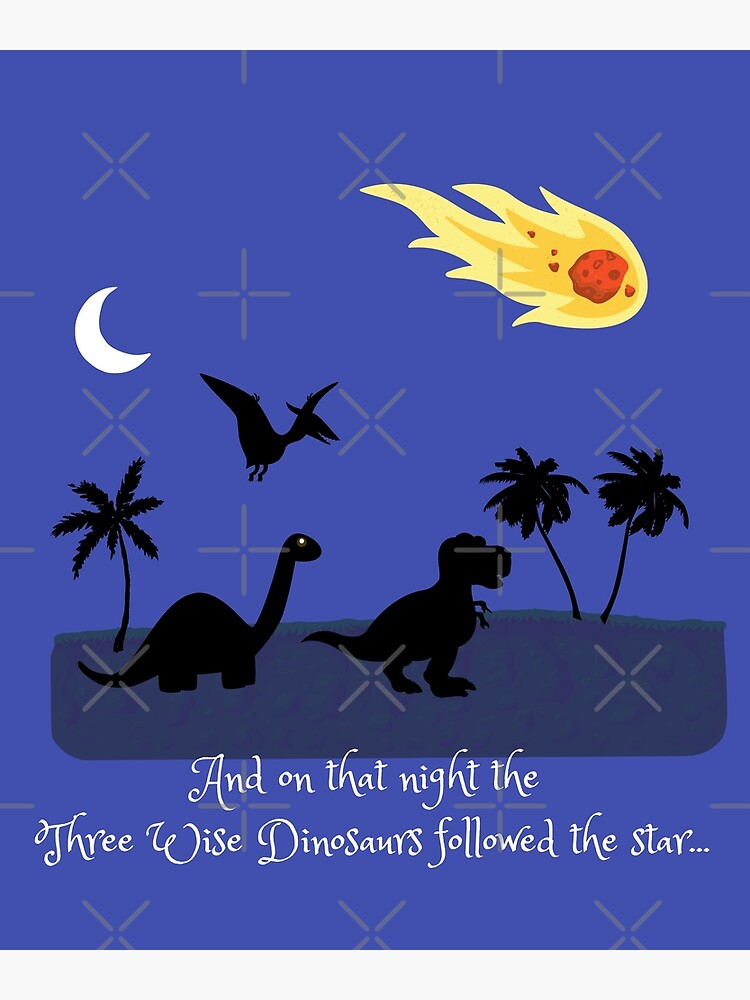The image is a vibrant, multi-colored graphic with a vertically rectangular layout and no border. The blue background is adorned with rotating silver Xs and plus signs, reminiscent of a watermark. At the very bottom, the text in white reads, "and on that night the three wise dinosaurs followed the star." Just above the text, a gray ground supports the black silhouettes of three dinosaurs: a Tyrannosaurus rex, a Brachiosaurus, and a flying Pterodactyl. Three palm trees in matching black—two in the foreground and one in the background—further decorate the scene. On the left side of the image, a crescent moon gleams, while on the upper right, a flaming meteor in orange and yellow streaks downward, suggesting a dramatic moment. This striking image evokes the whimsical and imaginative style often seen on card covers or children's book illustrations.